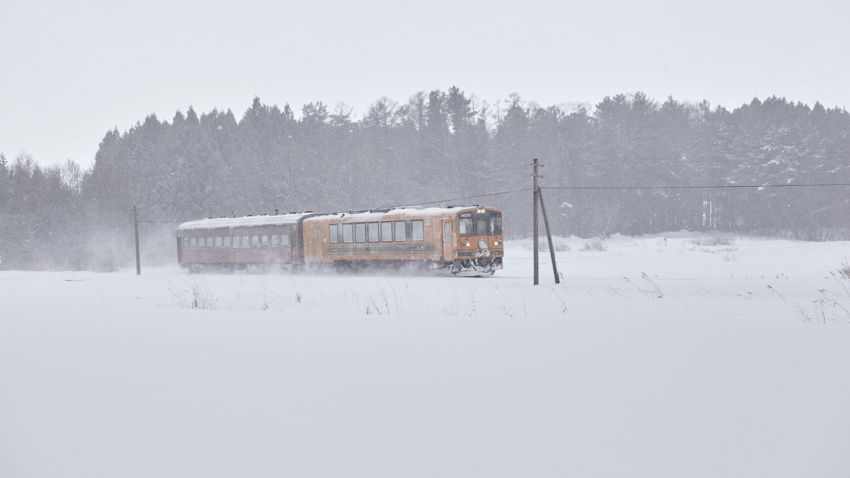This landscape photograph, taken during a snowstorm, features a striking scene dominated by the frosty grip of winter. A vibrant yellow train, with its headlights cutting through the snow, traverses the center of the image from left to right. The train consists of two cars: the front car is bright yellow with about seven gray-tinted windows and twin yellow headlights, while the rear car is a darker red, both capped with snowy roofs. Both cars have accumulated a layer of snow, enhancing their frosty appearance. Surrounding the train, the ground is completely blanketed in pristine white snow, broken only by the occasional tuft of grass struggling through the cold. Above, the sky mirrors the ground's whiteness, creating a cohesive, wintry panorama. In the background, a dense forest of snow-dusted pine trees stands in stark contrast to the vivid colors of the train. Overhead, a pair of power lines stretch between two poles, one of which is braced by another, faintly visible against the snowy backdrop. This vivid and detailed portrayal of a train in motion through a wintry landscape captures the tranquil yet powerful essence of a snowstorm.